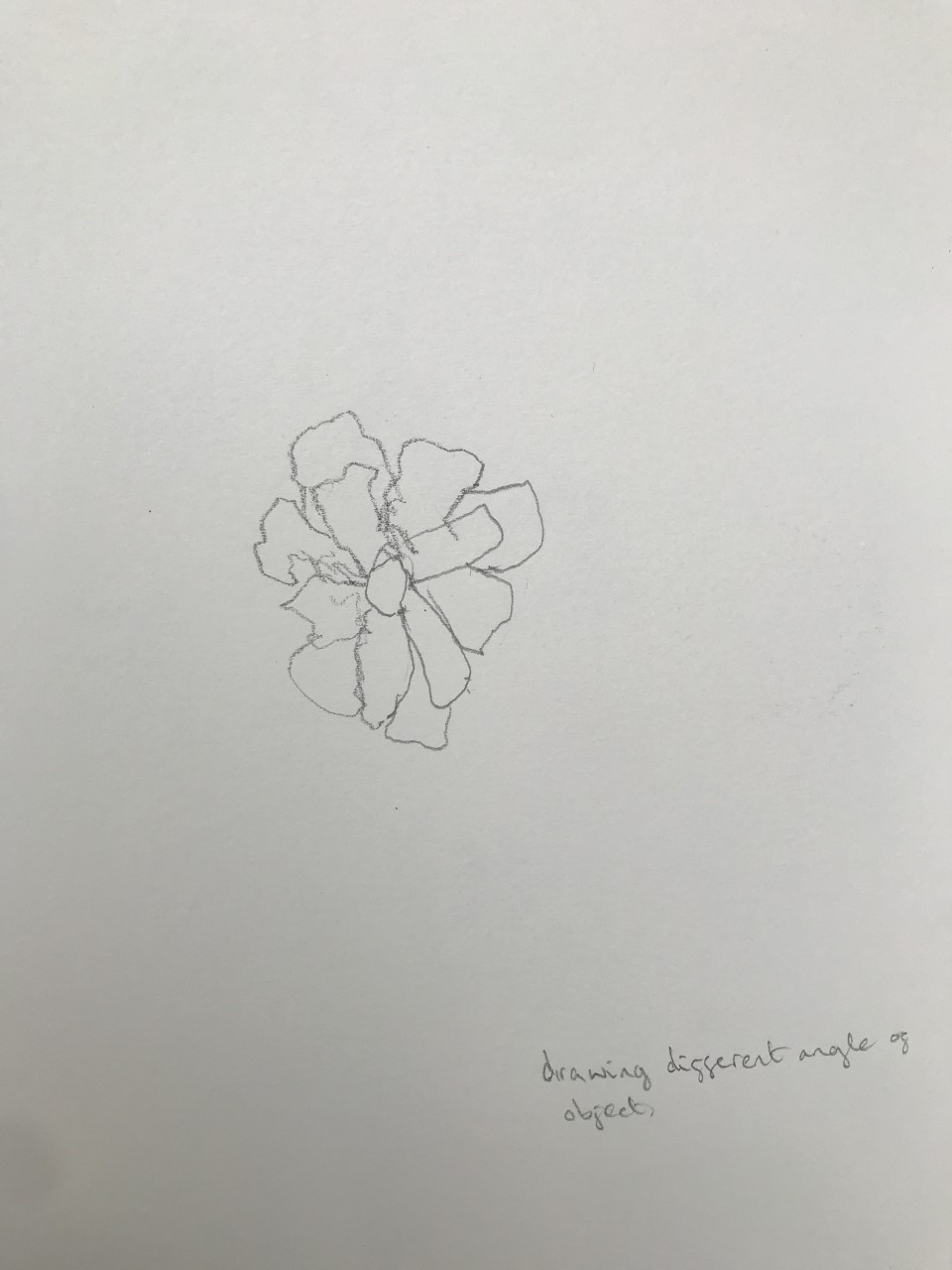This detailed caption describes an image of a drawing that resembles a flower. The illustration is rendered on white sketch paper and appears to be created by a novice artist or a child, characterized by its simple and imperfect lines. The flower is depicted with a circle at its center, surrounded by multiple layers of petals. 

The top layer consists of five distinct petals, while the bottom layer features seven petals, creating a sense of depth. Notably, a handwritten note in cursive pencil script is visible at the bottom right-hand corner of the sketch, reading, "drawing different angle of object." This adds an instructional element to the piece, suggesting an educational or practice context.